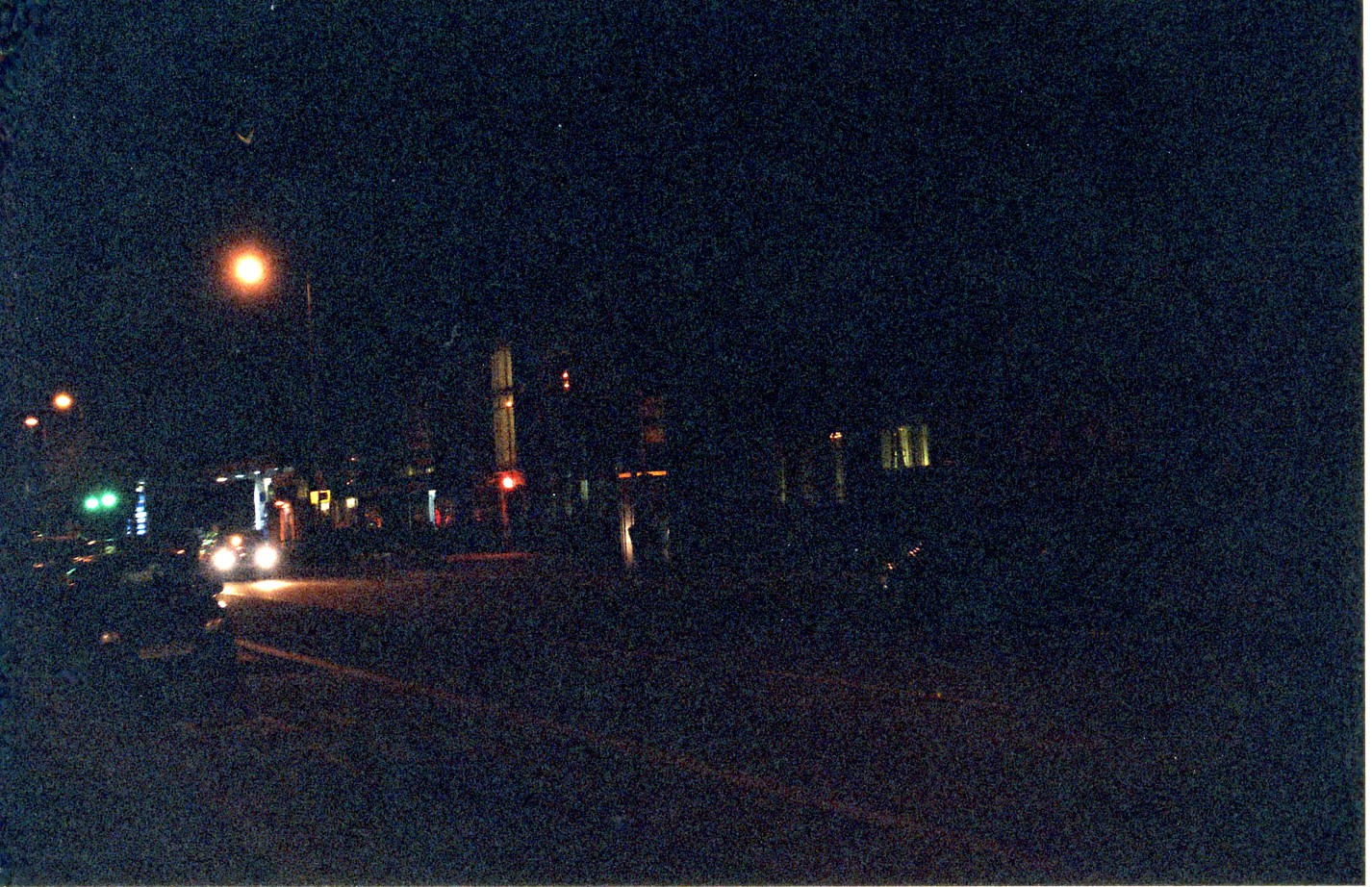A digital photo taken at night outdoors depicts a dimly lit, grainy urban street scene. In the foreground, a car with distinctly visible headlights is heading towards the viewer. The street appears to be lined with parked cars on both sides. The scene's left side reveals the end of a street stretching into the distance, framed by blurry streetlights casting yellow or greenish hues. Above and to the left, against the dark sky, a couple of green traffic lights hang suspended. The right side of the image shows several multi-story buildings in the distance, with various windows illuminated in yellow light, suggesting either homes or residential apartments. Among these buildings, closer to the street’s center but to the right, a brightly lit storefront possibly belonging to a gas station stands out. The overall scene is rendered with indistinct lines and details, characteristic of a night photograph taken with a cell phone.